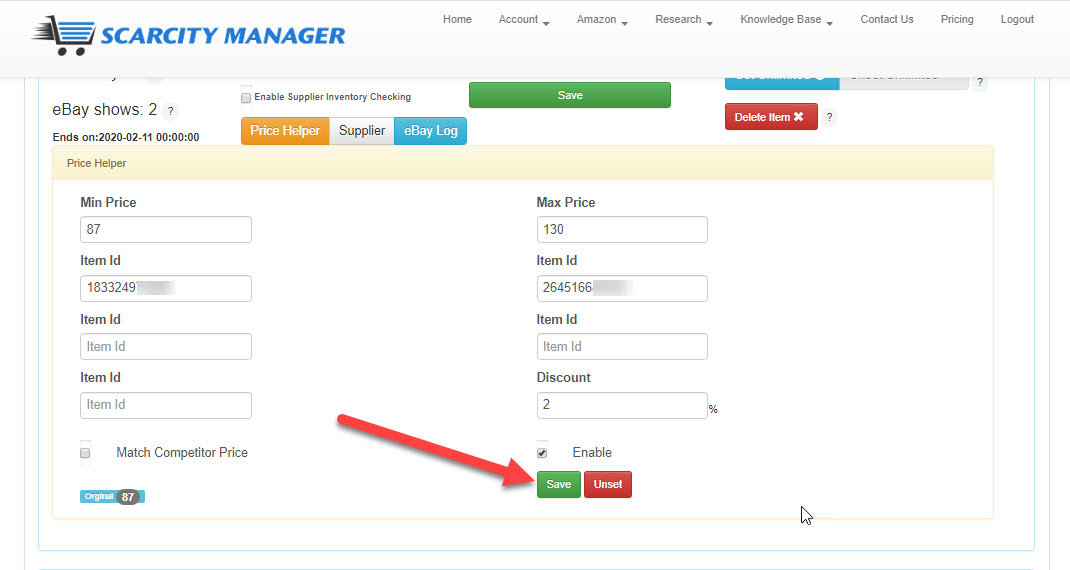At the top of the image, a gray rectangle features the title "Scarcity Manager" in blue letters. Adjacent to this text is an illustration of a shopping cart, depicted with visible wheels and trailing black lines to suggest rapid movement.

Below this header, a row of black text spans from left to right, reading: "Home," "Account," "Amazon," "Research," "Knowledge Base," "Contact Us," "Price," and "Logout."

Further down, the text "eBay shows two" introduces three horizontal rectangles arranged side by side. The first is orange with "Price Helper" written in white letters, the second is gray with "Supplier" written in black letters, and the third is blue with "eBay Log" written in white letters. 

Alongside these, there are additional colored rectangles: a green one labeled "Save" and a red one labeled "Delete Item." Below these is a light pink rectangle labeled "Price Helper."

The layout continues with several vertical columns. The first column lists "Min Price" and "Item ID" repeatedly, followed by "Match Competitor Price." The second column lists "Max Price" and "Item ID," followed by "Discount."

A red arrow points towards two rectangles in the second column. The first rectangle is green and says "Save," and the rectangle below it is red and says "Unset." Above these two rectangles is the word "Enable," accompanied by a small square with a black checkmark inside it.